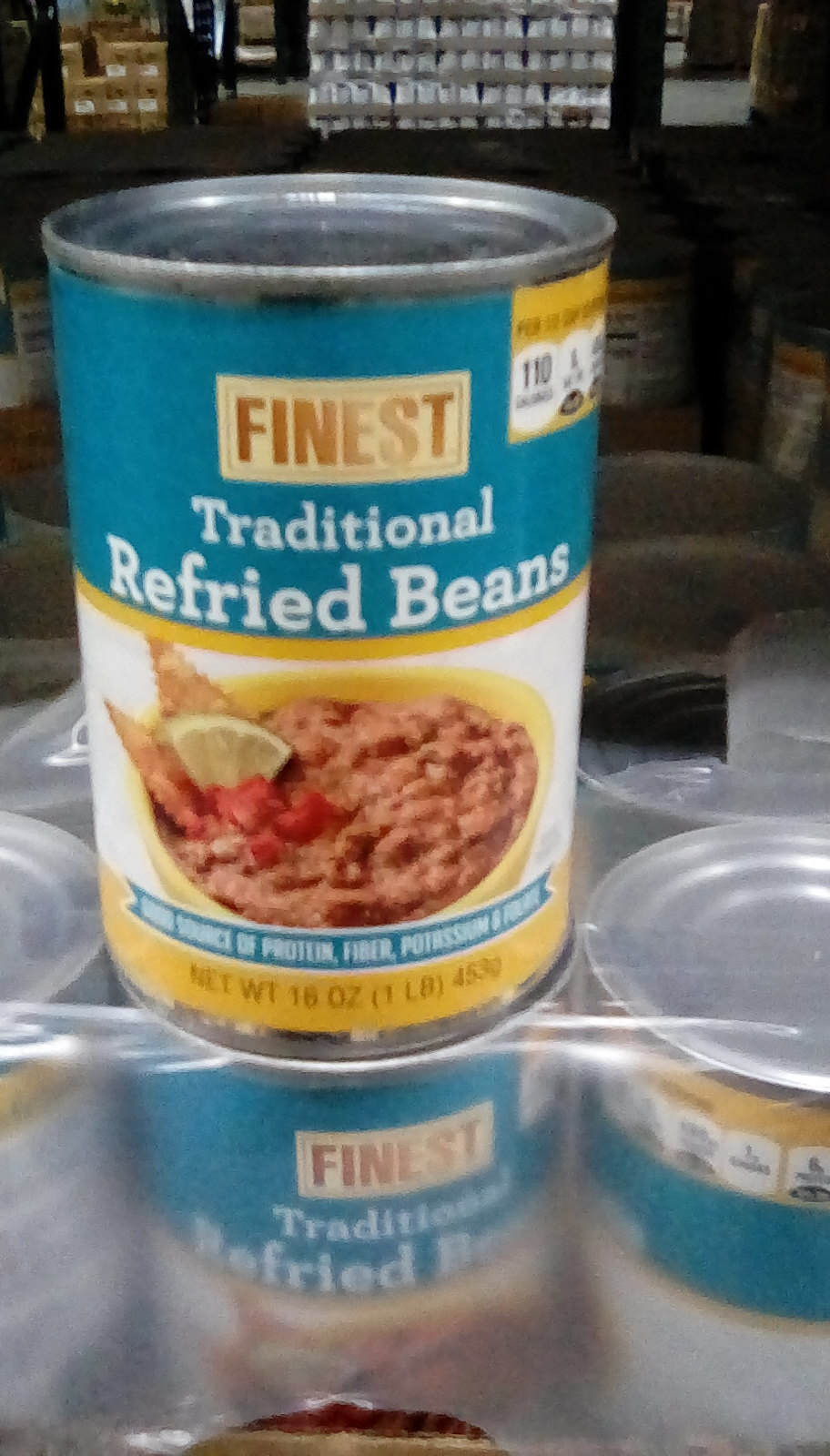The image depicts a tall can of "Finest Traditional Refried Beans." The can stands on the second shelf of a display, viewed slightly from above, allowing the top of the can to be visible. The label of the can is predominantly teal in the top third, transitioning into a white background, followed by a medium yellow strip at the bottom. The brand name "Finest" appears in gold. The can also advertises its nutritional benefits, stating it is a good source of protein, fiber, and potassium. There is a depiction of a yellow bowl filled with refried beans, a lime, and two tortilla chips in the upper left corner of the white section. The can's net weight is 16 ounces. The surrounding context suggests it is placed in a store setting, potentially as part of a promotional display.